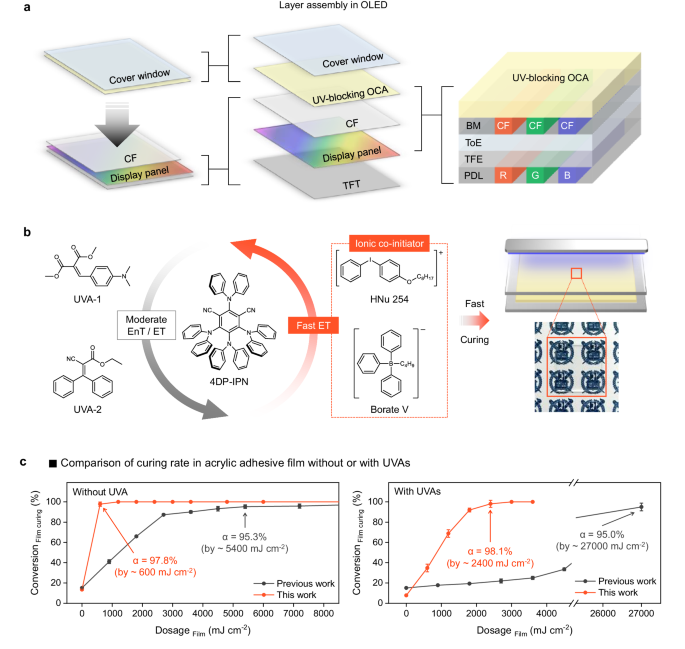This instructional diagram is divided into three sections: A, B, and C. At the top of the diagram, labeled as section A, we have a detailed layer assembly of an OLED. This section illustrates the step-by-step construction of the OLED display, starting with a cover window, followed by a UV blocking OCA, CF, display panel, and TFT layer. This portion also details the full assembly, listing components such as UV blocking OCA, BM, CF in red, green, and blue, TOE, TFE, and PDL for red, green, and blue layers.

In section B, the diagram presents a honeycomb pattern indicating two different compounds, labeled as UVA1 and UVA2, along with another compound, 4DP-IPN, surrounded by arrows indicating moderate and fast curing rates. There is also a red-bordered box indicating an ionic co-inhibitor with the compounds HNU254 and borate V, emphasizing the fast curing process with red arrows. 

Section C at the bottom features a comparison of curing rates in acrylic adhesive film with and without UVAs. The charts in this section compare the performance of current work (in red) and previous work (in black). Without UVAs, the current work shows a significant improvement, reaching nearly 100% conversion with a low dose, while previous work levels off around 80%. With UVAs, the current work again approaches 100% conversion, significantly outperforming the approximately 20% conversion observed in previous work. The charts clearly depict higher efficiency and improved curing rates with the use of UVAs by showing red lines above black lines in both scenarios, highlighting the substantial advancements made.